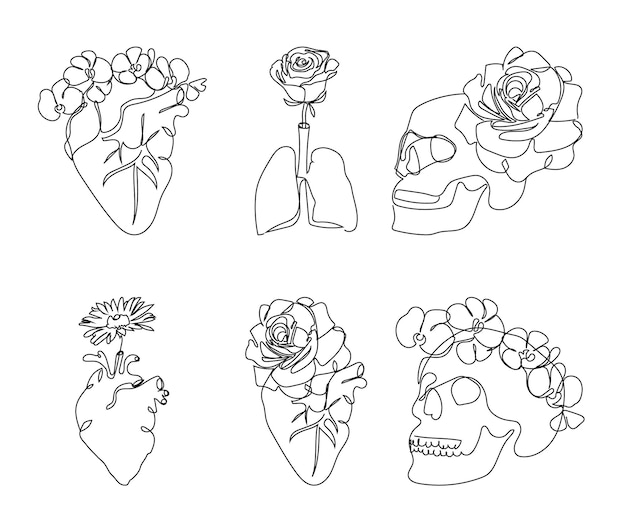The image showcases a collection of detailed, hand-drawn line art, all rendered in black and white without any coloring or shading. There are six distinct drawings arranged in two rows against a solid white background. Each row comprises three images that combine anatomical elements with floral motifs.

In the top row, starting from the left, there's an anatomically accurate heart with four flowers sprouting from its top. In the middle, a set of lungs is depicted with a rose emerging from the top tube, almost as if the lungs are being used as a vase. The third image in this row is a skull angled slightly to the left, adorned with a large rose on the side of its head.

Moving to the bottom row, the first image features another heart with a single flower growing from one of its top veins. The middle drawing presents a heart with a fully bloomed rose covering its top. The final image on the right is another skull, also facing slightly left, but this one is circled by a ring of flowers, resembling a floral crown.

Together, these drawings create a striking juxtaposition of human anatomy and delicate floral elements, emphasizing the blend of life and decay, while offering potential for further artistic interpretation through coloring.